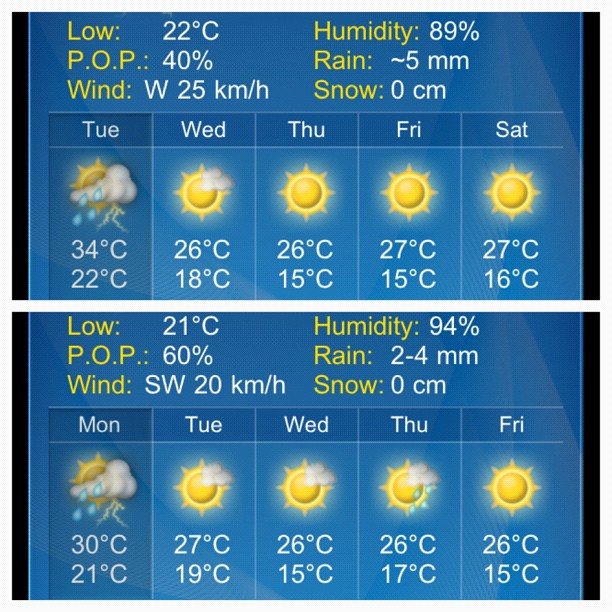The image depicts two detailed weather forecasts side by side, each presented against a traditional blue backdrop typical of weather apps, complete with sunny symbols and temperatures denoted in white text alongside weather markers in yellow text. 

The top forecast lists a range of weather details: a low of 22 degrees Celsius, a probability of precipitation (POP) at 40%, westerly winds at 25 kilometers per hour, 89% humidity, and rainfall up to 5 millimeters with no snow accumulation. The weekly forecasts show highs between 34 and 27 degrees Celsius: Tuesday (34/22), Wednesday (26/18), Thursday (26/15), Friday (27/15), and Saturday (27/16).

The bottom forecast includes slightly different details: a low of 21 degrees Celsius, a higher POP at 60%, southwesterly winds at 20 kilometers per hour, 94% humidity, and rainfall between 2 to 4 millimeters with no snow expected. The projected daily temperatures are: Monday (30/21), Tuesday (27/19), Wednesday (26/15), Thursday (26/17), and Friday (26/15).

Both forecasts provide comprehensive weather conditions, aiding in planning for the upcoming days.